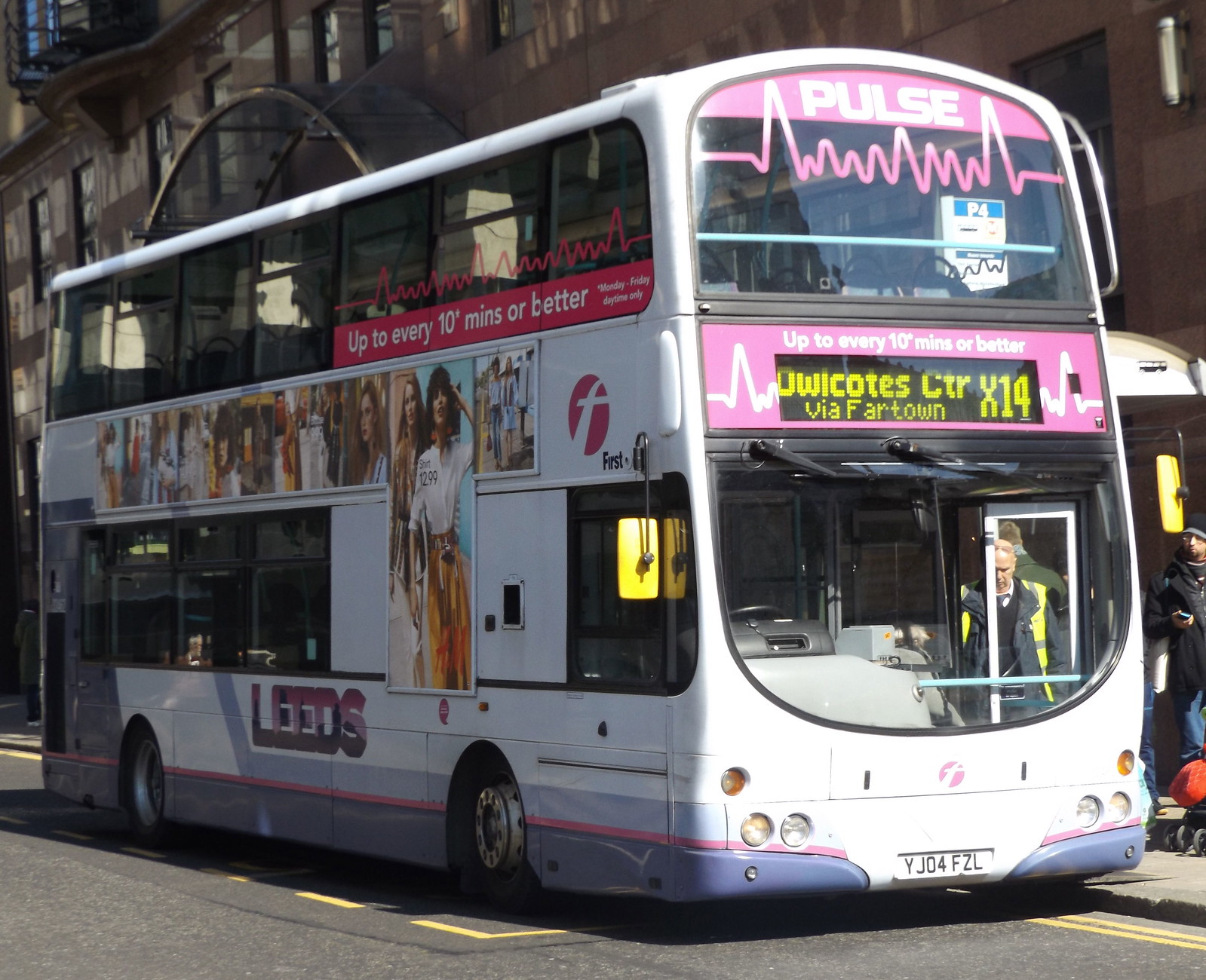This photograph captures a vivid scene in the city of Leeds, featuring a double-decker bus at a bus stop on an asphalt street. The bus, painted primarily white with distinct pink detailing at the very top of the windshield, is a recognizable vehicle with the branding "PULSE" and a heartbeat graphic prominently displayed. Below this, in pink, is the promise "up to every 10 minutes or better."

In the midsection of the windshield, a yellow insert provides route information, indicating "OWICOTES CTR" (Owlcote Centre) and "X14 via FARTOWN." The driver, wearing a black jacket with yellow suspenders, appears to be in the process of getting onto the bus, highlighting a moment of transition.

Adding to the visual interest, the side of the bus features a large advertisement for a women's clothing store. This ad showcases two full-sized images of women: one model in a white shirt paired with orange pants, and another donning a khaki shirt with white pants. The ad emphasizes the fashionable appeal of the store's offerings.

On a sunny day, the bus is stationed near a building characterized by numerous windows and brickwork. A person stands nearby, waiting to board, in a black jacket, black hat, jeans, and accompanied by a red bag on a trolley. Additionally, the bus carries the license plate YJ04FZL, further cementing its identity within this urban setting.